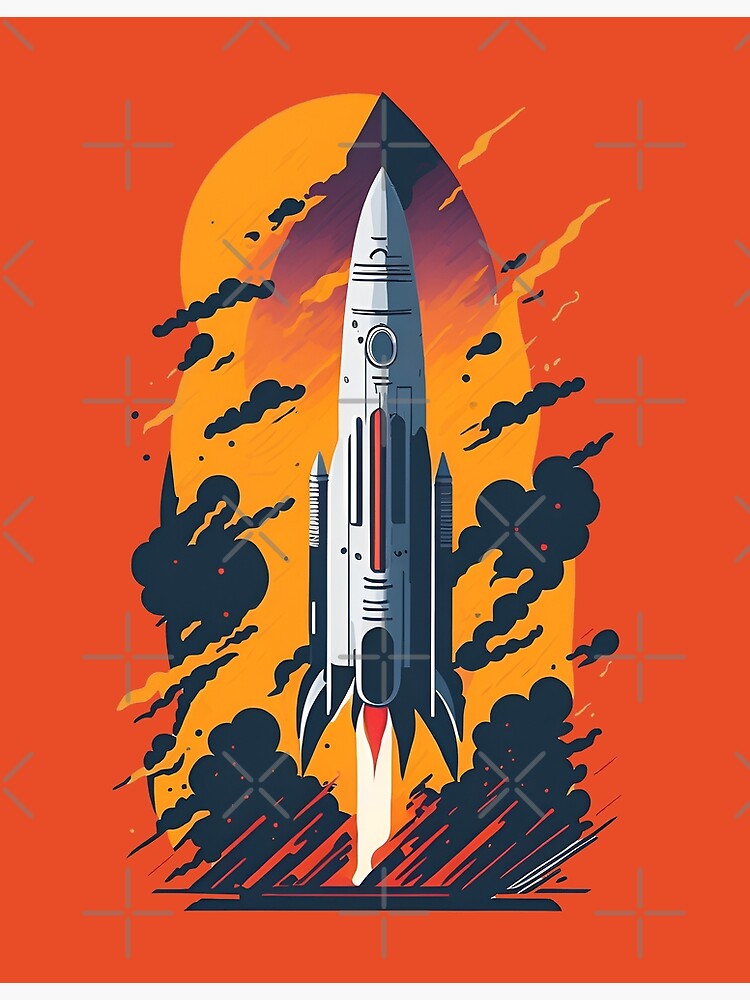The vertically oriented poster features a dark orange background with an array of digital crosshairs and plus signs in light gray. Centered in the image is a large, pointed rocket ship with an oval window at its top and an orange stripe running down its center. The rocket, primarily whitish-gray, is depicted launching upward amidst billowing black clouds, some with red dots and holes. Beneath the rocket, flames and fiery trails extend downward, suggesting it is some distance from the ground, which is represented by a thick black horizontal line. On either side of the central rocket are two smaller missile-like boosters. The background creates a dramatic effect with dark yellow highlights around the rocket and the presence of a yellow sun and additional stars, enhancing the clean and dynamic aesthetic of the poster.